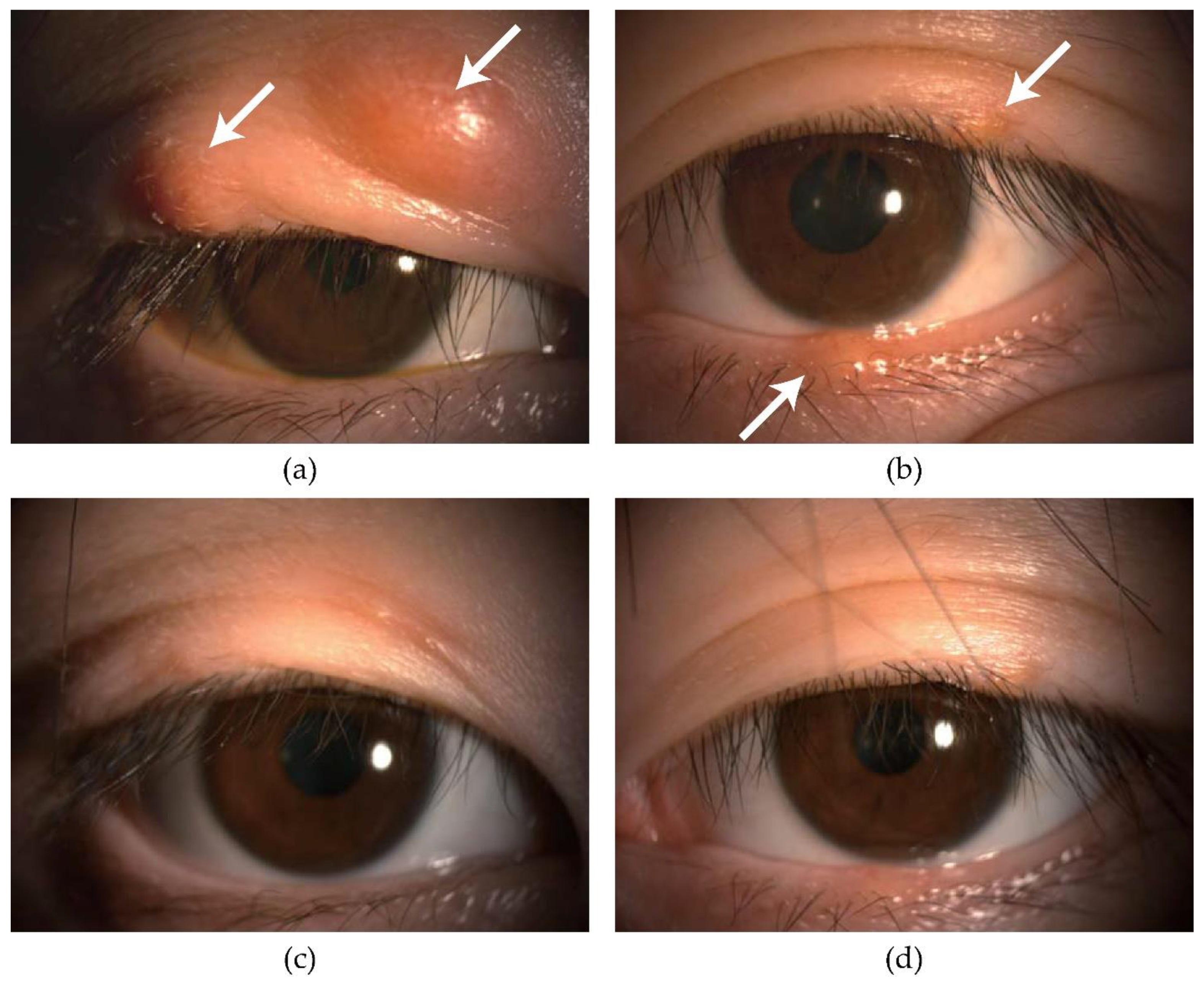The image is a detailed close-up collage of four photographs of a person's eyes arranged in a 2x2 grid, labeled A, B, C, and D beneath each image within white brackets. Photograph A, in the upper left, shows a brown eye with significant swelling on the upper eyelid, characterized by two reddish lumps to which white arrows point, indicating the areas of concern. Photograph B, in the upper right, also portrays a brown eye but with less pronounced swelling, showing smaller raised areas on both the upper and lower eyelids, each marked by white arrows. Photograph C, in the lower left, depicts the same brown eye as A, now appearing normal with no swelling or arrows indicating issues. Similarly, Photograph D, in the lower right, shows the same brown eye as B, significantly healed with only a faint remnant of swelling on the upper eyelid, and no issues on the lower eyelid. The consistent fair skin and brown hair in the images suggest they belong to the same individual, showing the progression of an eye condition from its worst state to nearly full recovery.